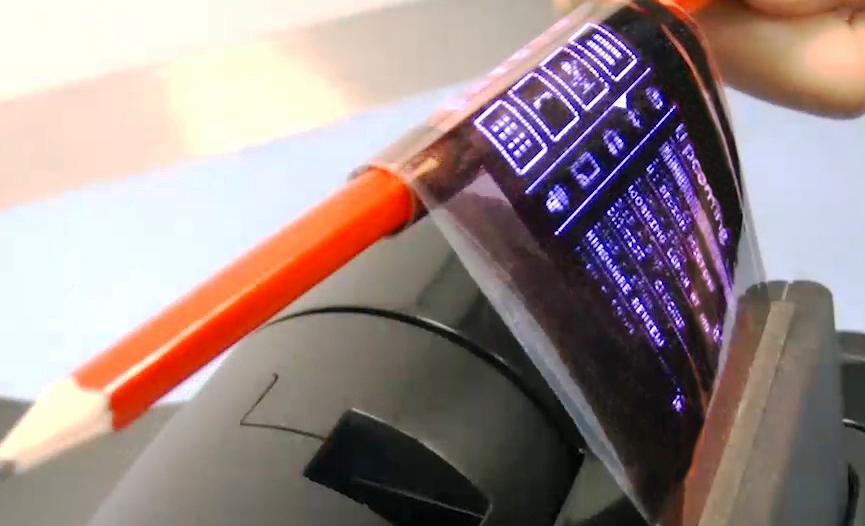In this close-up image, a sharpened red-orange pencil, positioned diagonally from the top right to the bottom left, is being intricately wrapped in a strip of thin black plastic film, reminiscent of camera film or receipt paper. The plastic film, which extends from a gray, receipt-like contraption at the bottom of the image, features blue writing against a dark background, including icons and the word "upcoming" that evoke a digital interface. A hand is visible in the top right corner, delicately guiding the pencil as it rolls the film, showcasing a fusion of traditional and modern elements.